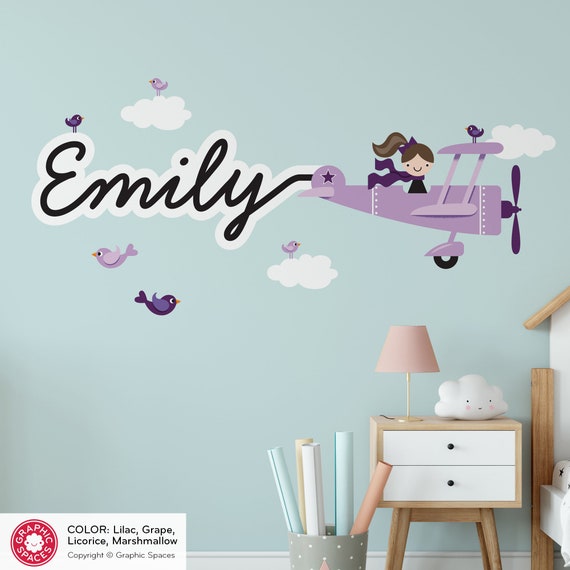The image features a meticulously decorated little girl's bedroom, primarily showcasing a pastel-hued wall that appears to be a soft, pale blue or sea foam green. Prominently, "Emily" is written in cursive black text with a white outline, creating a whimsical touch. The mural includes a cartoon drawing of a smiling little girl with a brown ponytail and a purple bow, flying a lilac-colored airplane with a star on its tail. She wears a dark purple scarf that flutters behind her, portraying mid-flight action. Puff-like, white clouds populate the background alongside various shades of purple birds, adding to the dreamlike quality of the room.

The wall acts almost like a canvas for a sky scene, with three puffy clouds and cartoonish purple birds oriented both left and right. To the bottom right, there is a nightstand made of wood with white drawer fronts, hosting a pink-shaded lamp and a puffy cloud-shaped lamp, emphasizing the room's cohesive theme. The bedding is seen partially, showing a white fabric adorned with blue stars, enhancing the serene nighttime atmosphere.

Additionally, the design details include a white box with text at the bottom corners, marked by the words "Graphic Spaces" and specifying the color scheme: lilac, grape, licorice, and marshmallow, with a clear copyright notice indicating that this is part of a Graphic Spaces collection.